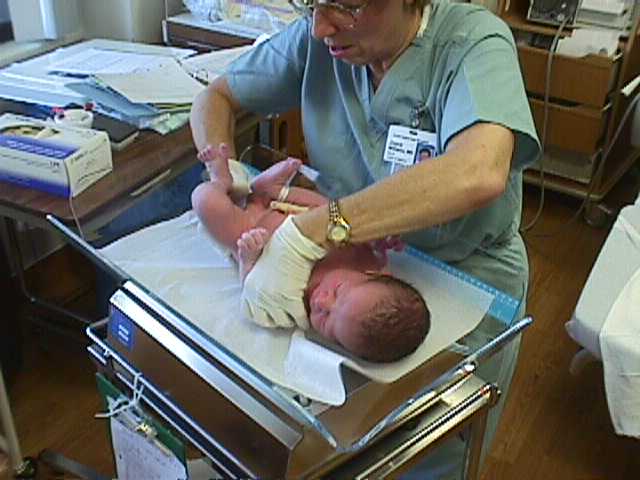The image depicts a newborn baby being attended to by a nurse in a hospital room, likely a neonatal ward. The newborn, naked with dark, slightly curly hair, is placed on a glass-like weighing scale. The nurse, clad in a light green nursing outfit and white gloves, is delicately handling the baby, with one hand on the infant's shoulder and the other near the groin. She has a white name tag clipped to her chest and is wearing a gold watch. The room is clearly a medical setting with a tidy, albeit busy, arrangement. Behind the nurse, there is a brown cart with various wires extending from it. To the left, a brown table holds a box of latex gloves and scattered papers, illuminated by daylight streaming through a window. On the right, one can observe the corner of a hospital bed with a white fitted sheet and a white blanket draped over the edge. The floor appears to be hardwood, contributing to the overall tranquil atmosphere of the room.